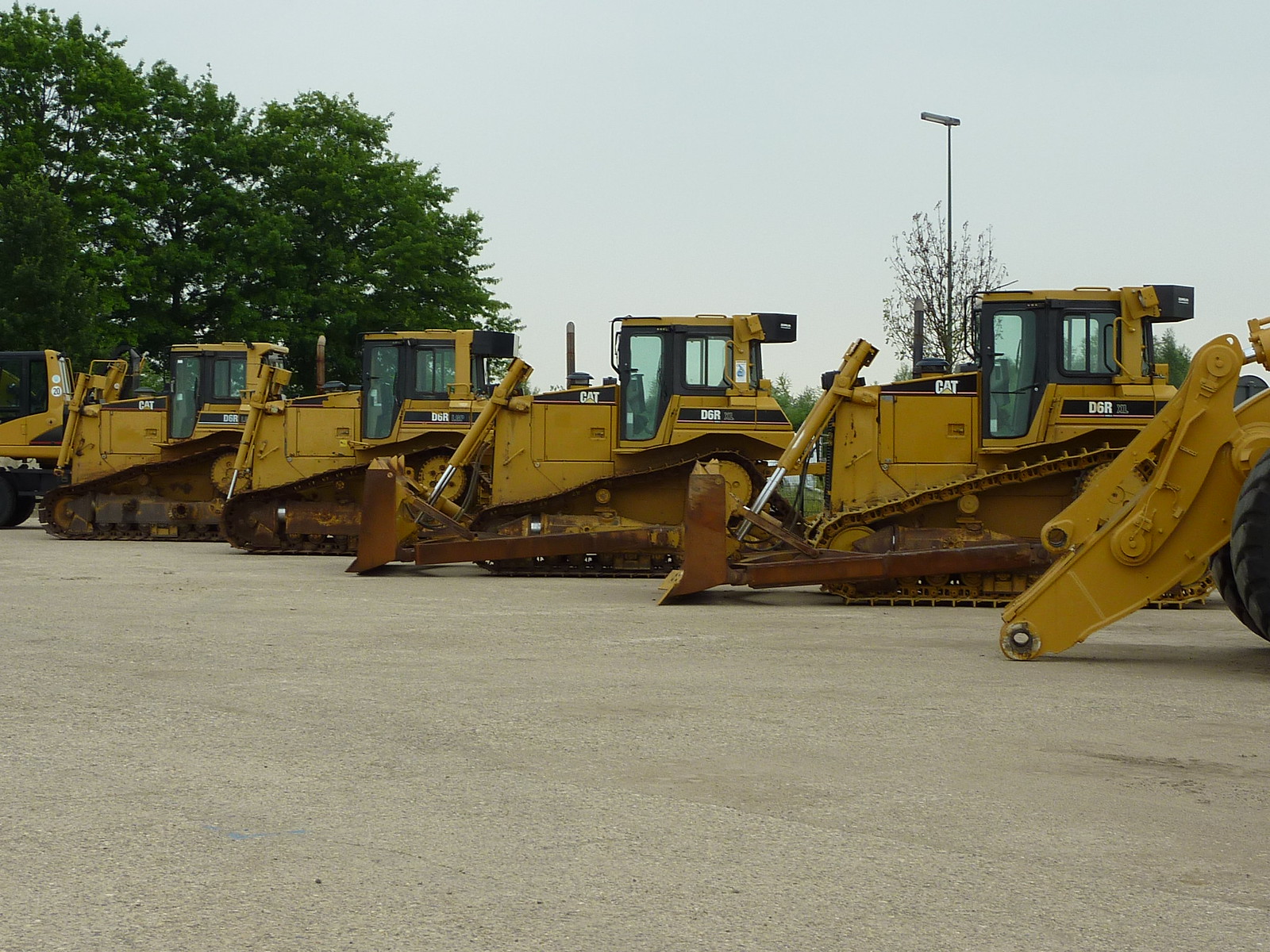This color photograph captures a lineup of five CAT brand heavy machinery, predominantly bulldozers, parked on an asphalt lot under an overcast, light gray sky. The machinery, characterized by their orange bodies with black trim and enclosed cabs, are arranged at an angle from right to left, facing slightly away from the viewer. Each of these bulldozers has its blade lowered and is equipped with high roller tracks. Just visible at the right edge of the frame are the arms of a sixth piece of equipment with wheels. The background features tall deciduous trees on the left side and a streetlight standing near the center-right, next to a small skinny tree with sparse leaves. The photograph emphasizes the idle strength and orderly arrangement of these robust machines.